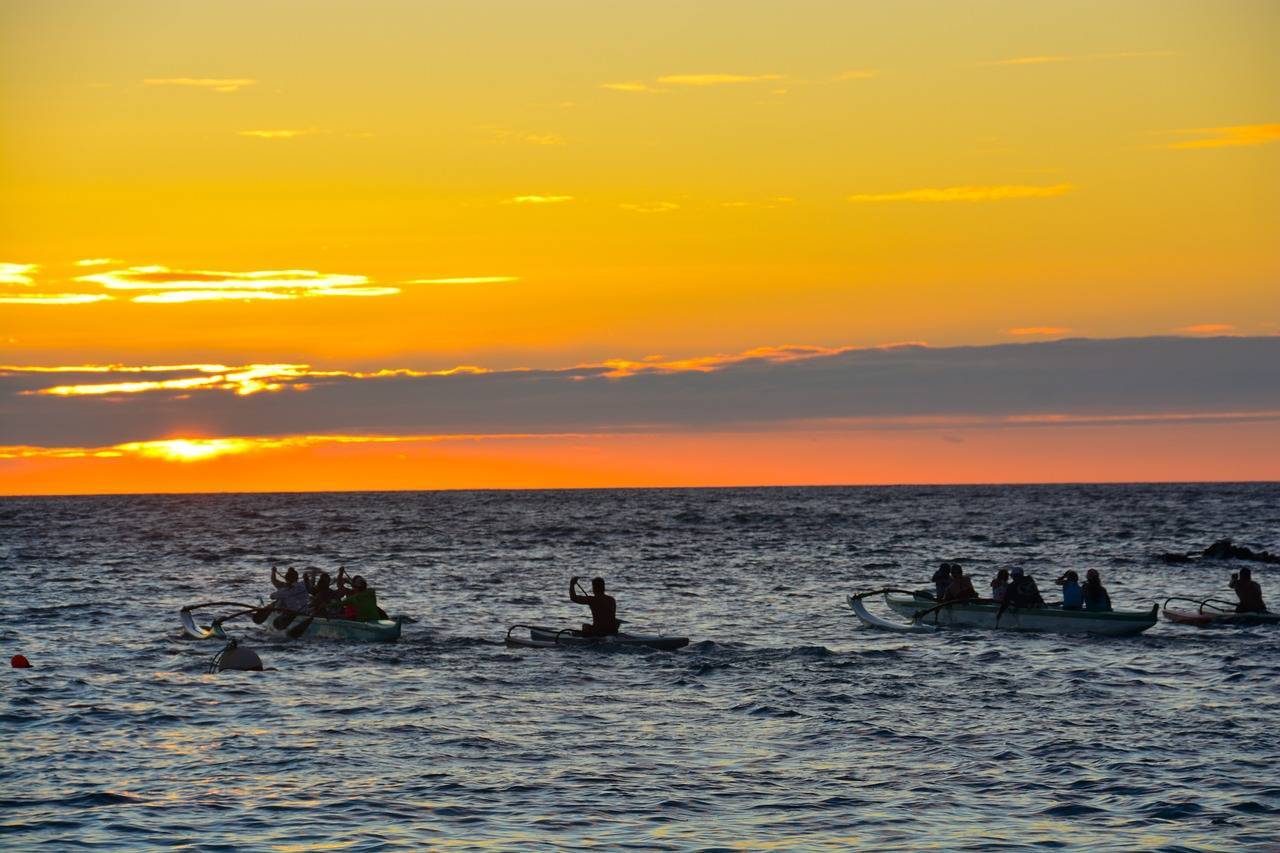This captivating photograph, taken outdoors on the ocean during a sunset, showcases a serene yet vibrant setting. The image is beautifully split, with the lower half dominated by the tranquil, vast expanse of water, and the upper half by an enchanting sky. The sky transitions smoothly from a light blue at the top, through a gradient of orange, down to a yellow hue, crowned by the sun partially hidden behind a stretch of gray clouds on the left-hand side.

Positioned from left to right, the silhouette of a boat loaded with people, supported by twin pontoons, stands out. Next, towards the middle, a lone rower pilots a small boat. Just behind this, another twin-hulled boat carrying around six people can be seen. The silhouettes of the individuals, engaged in rowing, add a subtle narrative of motion and effort. A bit further behind, another single-person boat completes this harmonious maritime scene. The lack of textual details keeps the focus entirely on the essence of the natural beauty and the interaction of humans with their environment during this magical twilight moment.